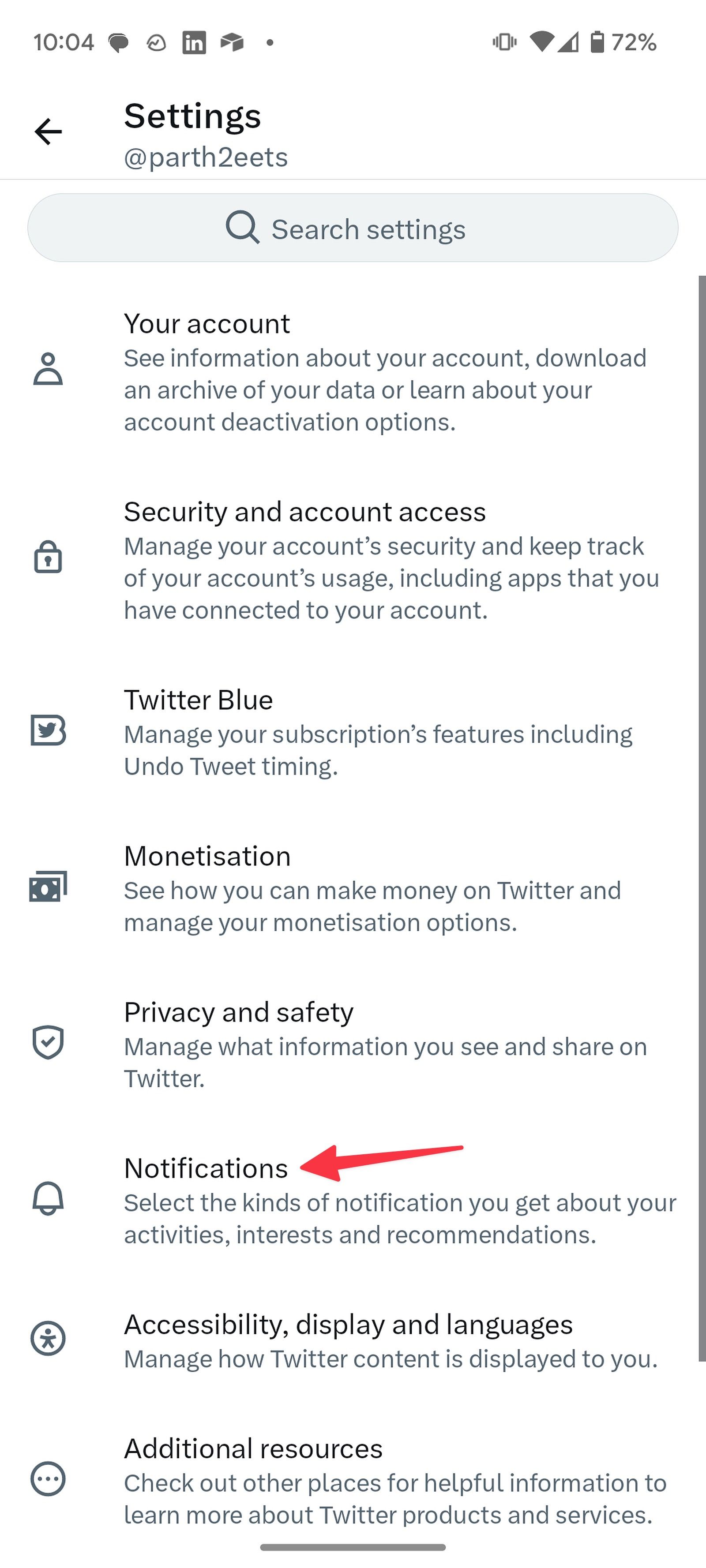In the image, we see a screenshot of a smartphone's settings list, displayed on a white background with gray text in the upper left corner. At the top, the time is shown as 10:04 AM, and on the far right, a battery icon indicates a 72% charge. An arrow pointing to the left and the word "Settings" are visible at the top, followed by the header "PARTH 2EETS". Below this header, there's a gray search bar labeled "Search settings".

Immediately underneath the search bar is a vertical list of settings options, each accompanied by an icon. 

1. **Your Account** (Person icon): This section allows you to see information about your account, download an archive of your data, or learn about deactivation options.
   
2. **Security and Account Access** (Padlock icon): Manage your account's security and keep track of your account's usage. It also includes downloading apps connected to your account.

3. **Twitter Blue** (Twitter icon): Manage features of your Twitter Blue subscription, including the timing for undoing tweets.

4. **Monetization** (Dollar bill icon): Explore methods for making money on Twitter and manage your monetization options.

5. **Privacy and Safety** (Shield with check mark icon): Control the information you see and share on Twitter to enhance your privacy and safety.

6. **Notifications** (Bell icon with a red arrow): Customize the types of notifications you receive about your activities, interests, and recommendations.

7. **Accessibility, Display, and Languages** (Circle with a person icon): Adjust settings related to accessibility, display preferences, and language options.

8. **Additional Resources** (Circle with dots icon): Access other available resources for additional support and information.